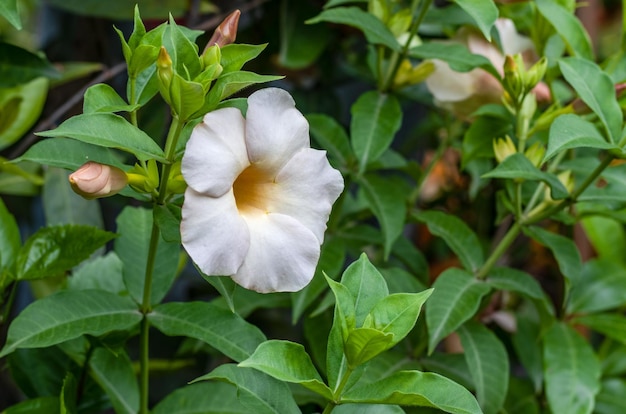This image captures a close-up of a white flower potentially identified as a hibiscus, which is prominently featured surrounded by medium to light green, glossy, pointed leaves. The flower has five petals encircling a distinct, slightly sunken yellow center. Flanking the main flower are several budding flowers, distinguishable by their light pinkish tinge. The photograph, focused precisely on the central flower, exhibits a shallow depth of field, rendering the background—a dense array of leaves and potentially additional white flowers—blurred. The overall lighting suggests an outdoor setting, enhancing the vividness and clarity of the primary subject against the softer, more diffused backdrop.